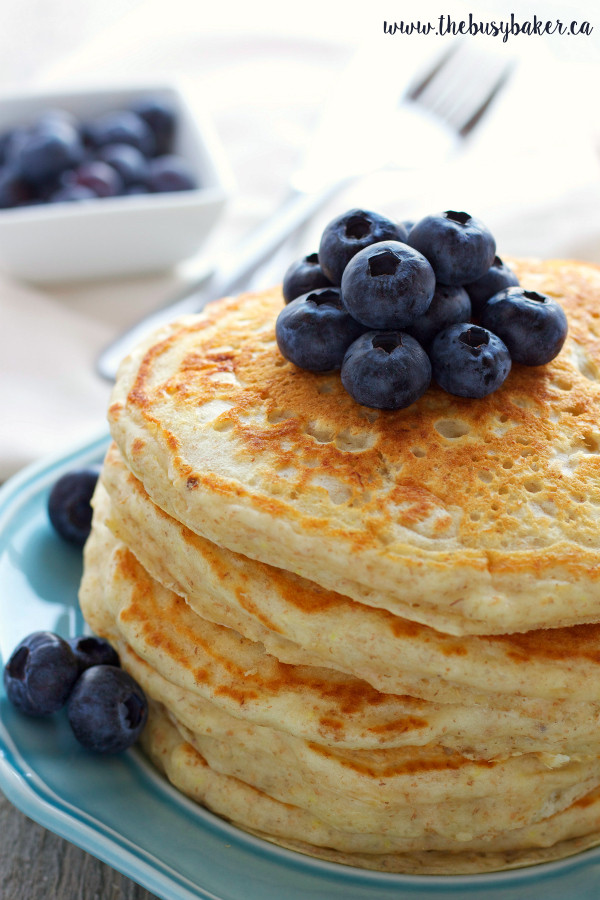This professional photograph captures a mouth-watering stack of five golden-brown pancakes, artfully displayed on a teal plate with a delicate line design near its edge. The pancakes, slightly uneven in texture, showcase enticing grill marks that emphasize their perfectly cooked surface. Atop the stack sits a generous pile of dark, plump blueberries, with a few more casually scattered on the plate to the left. The scene is set against a cream-colored tablecloth, creating a warm and inviting backdrop. The background features a blurry, washed-out depiction of a white, rectangular ceramic bowl filled with blueberries, accompanied by a similarly indistinct fork, all contributing to a sense of depth and context. This detailed composition highlights the appealing contrast between the light, fluffy pancakes, the deep blue of the blueberries, and the subtle teal of the plate.